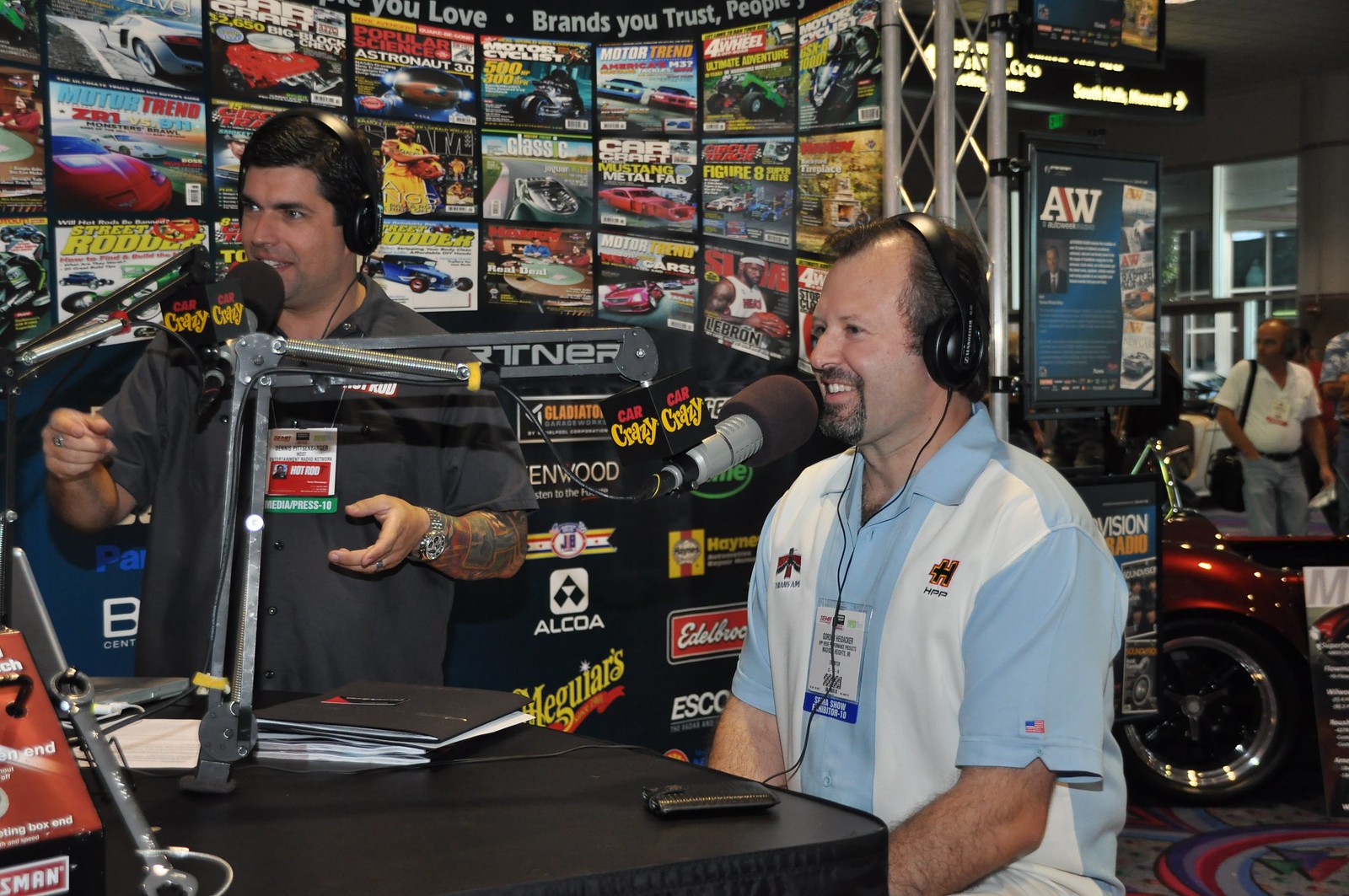In this indoor image taken in landscape mode, we see a bustling scene centered around a recording setup prominently positioned in the middle-left of the frame. A desk cluttered with various objects like a wallet, several books, a computer, some tools including a Craftsman wrench, and a couple of microphones extends from the bottom left corner. Two men, both wearing over-the-ear headphones, are engaged in a radio recording session. 

The man on the right, who is seated, is of Caucasian descent with a small beard and mustache. He wears a light blue and white striped short-sleeved collared shirt. The man to his left, who is standing, has a slightly darker complexion, sports tattoos on his arms, and is wearing a short-sleeved gray shirt. He is actively talking into his microphone, gesturing with his hands. 

Behind them, a black wall adorned with various car magazine covers, including titles such as Car Craft, Popular Science, Motorcyclist, Motor Trend, Four Wheel, Circle and Track, and Street Rotter, adds to the automotive theme. The microphones in front of them are labeled "Car Crazy," indicating the nature of their discussion. Additionally, sponsorship logos such as Meguars and Alcoa can be seen on the wall.

To the right side of the frame, the image transitions into an open auditorium or hallway where cars are on display. Several people can be seen walking around, examining the vehicles. The scene is alive with vibrant colors, including red, white, silver, black, blue, light blue, orange, and yellow, enhancing the dynamic atmosphere of what appears to be a car dealership, parts store, or auto show.